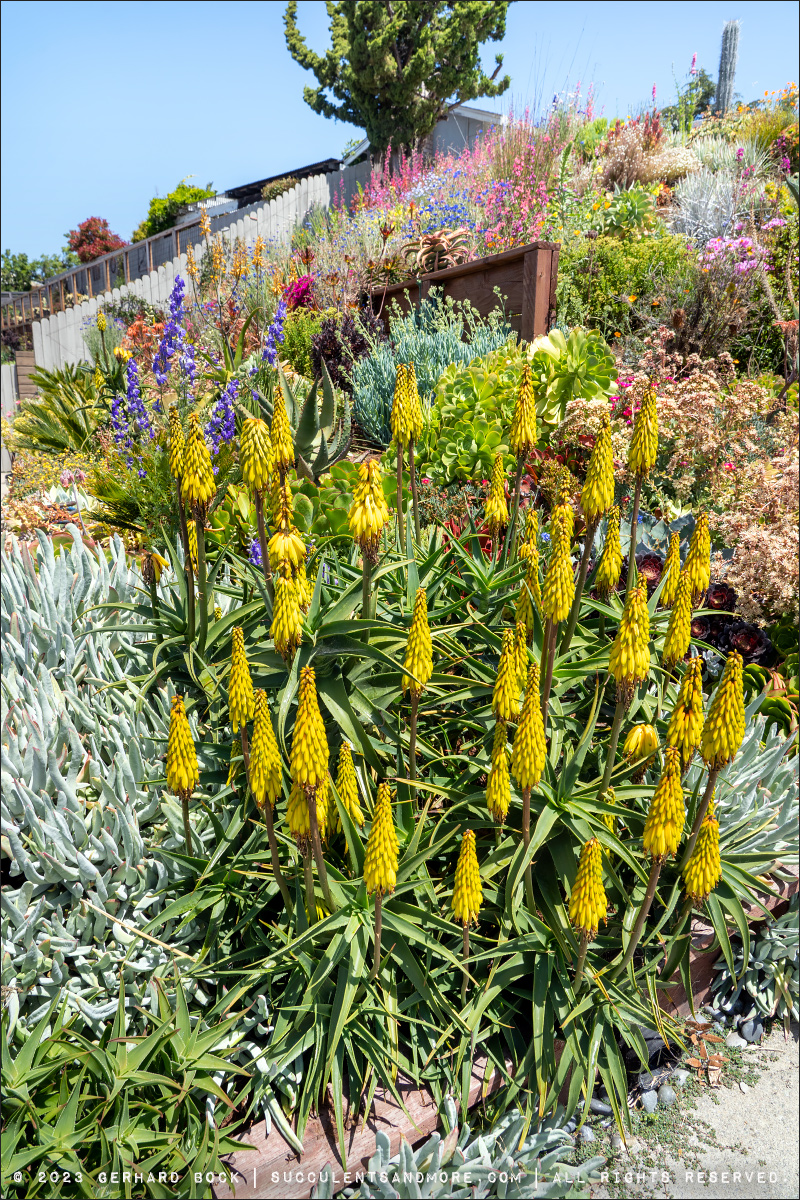The image depicts a vibrant hillside garden bathed in daylight, with a glimpse of blue sky and the rooftops of houses peeking out at the top. The garden is a riot of colors, teeming with blooming flowers and various greenery. Prominently in the foreground, there are striking yellow cone-shaped flowers resembling pineapples, with long, blade-like green leaves. Scattered throughout the garden are an assortment of flowers, including clusters of blue gladiolas and a mix of pink, light blue, and lavender blossoms. The foliage varies in both height and texture, from small shrubs to taller plants. Some descriptions mention the presence of bushes, some flowering and some just green, along with a fence and even a cactus at the top of the hill, indicating the arid nature of the area. The varied vegetation and colorful blooms create a captivating, almost wild garden scene on this hillside.